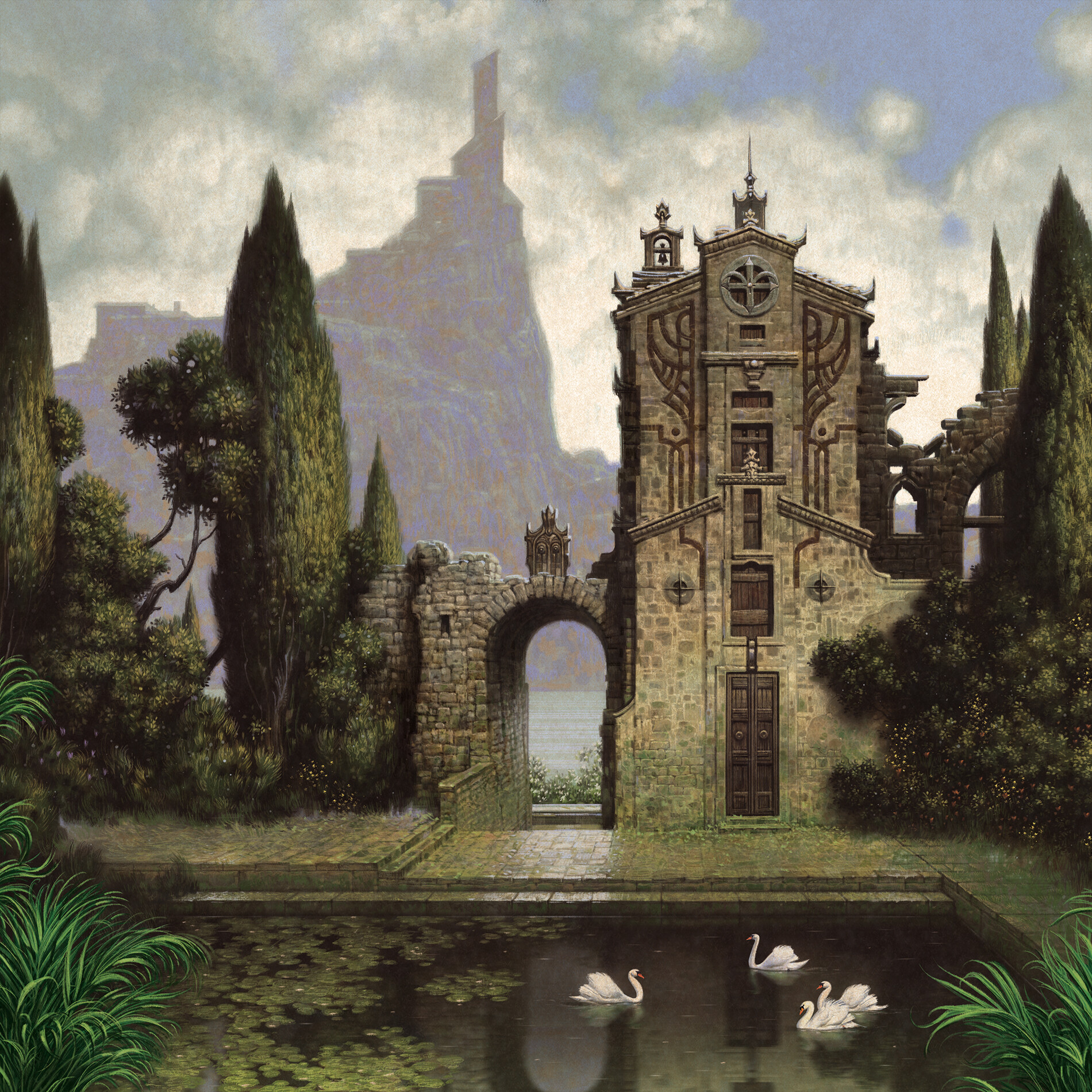This detailed painting captures a serene pool scene nestled in front of a grand gray stone building. The imposing structure towers above, flanked by a prominent stone arch on its left side. To the right, a bush and a tree provide a touch of greenery, with the top of another, taller stone arch peeking out in the distance beyond the tree. The left-hand side is bordered by a variety of trees, some towering and pointed while others are adorned with round clusters of leaves at their tips.

In the foreground, framing the scene, grass-like leaves or fronds with gentle curves are positioned at the lower left and right corners. The pool itself is square with dark, reflective water. On the right side of the pool, four elegant swans glide gracefully; three are heading left, while one swims in the opposite direction. To the left, lily pads or similar aquatic vegetation decorate the water's surface. The pool mirrors the surrounding architecture, capturing the stone arch and the building's window or door in its reflection.

Above and beyond the stately structure, the sky is a blend of blue and white clouds, setting a tranquil backdrop. The distant, foggy silhouette of a cliff or mountaintop adds depth and a touch of mystery to this idyllic landscape.